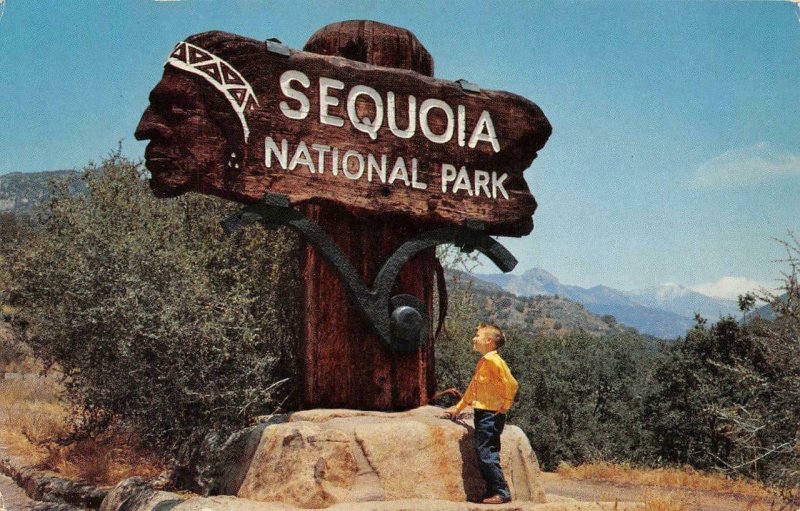This vintage photograph, likely from the 1950s or 60s, captures a bright, sunny day at Sequoia National Park. The focal point is an impressive, large wooden sign made from thick, dark lumber, possibly sequoia wood. The sign, in the shape of a wishbone mounted on a large flat rock, reads "Sequoia National Park" in white letters. Carved into the left side of the sign is an intricate profile of a Native American head, adorned with a headdress and earrings, looking to the left with a serious expression. 

A small boy with short blonde hair stands in front of the rock, gazing up at the sign. He is dressed in a long-sleeved bright yellow shirt, blue jeans, and boots, typical attire for the era. The background features clear blue skies with a few white clouds, a dense line of trees and foliage, and majestic mountain ranges in shades of green, blue, and gray. This idyllic scene encapsulates the timeless beauty and historic charm of Sequoia National Park.